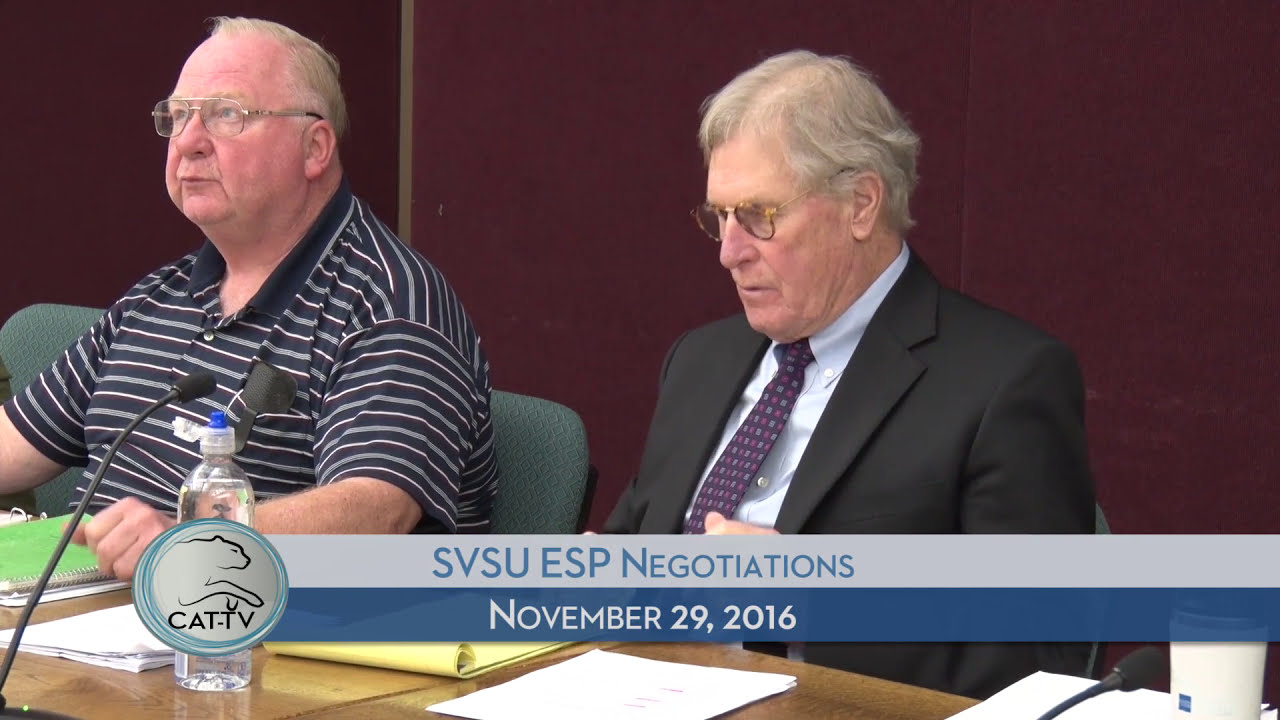The photograph shows two older white men sitting at a wooden table, likely in a political or committee meeting setting. Both are wearing glasses and seated on green office chairs. The man on the right is dressed formally in a black suit with a navy and red tie and light blue shirt; he has gray hair and a composed demeanor. In contrast, the man on the left is dressed more casually in a dark and white striped polo shirt, and has a red face, indicating probable health issues. He also has gray hair and is morbidly obese. On the table, there are various items including a water bottle and a black microphone in front of the man on the left, as well as a green notebook and a yellow legal pad near his elbow. The man on the right has a stack of white papers in front of him. The background appears to be purple. The image features an overlay text at the bottom corner reading, "SVSU ESP Negotiations" and "November 29th, 2016," with a silvery circular disc showing a depiction of a cat underneath text that reads "Cat TV."